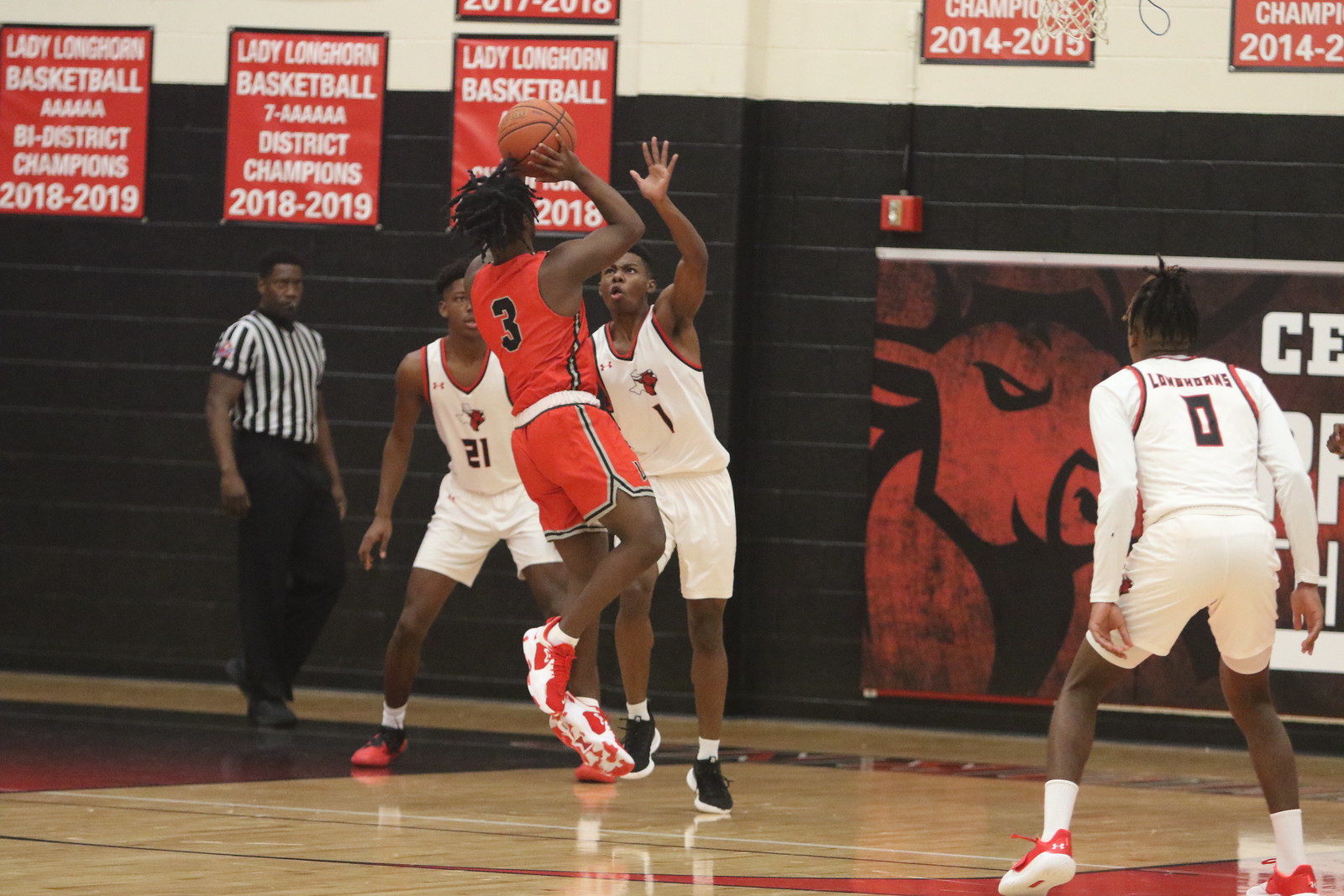In this detailed photograph taken inside a gymnasium in Doris, an intense basketball game is underway between two teams. The team in white jerseys, bearing the logo "Lady Longhorn Basketball" on their backs, features players numbered 0, 1, and 21. The player on the far right, number 0, is in an all-white uniform. Two more teammates, numbered 1 and 21, are positioned next to him. They are attempting to block an airborne player in a red jersey, number 3, who is about to shoot the basketball. This dynamic moment is captured with the red-jerseyed player's jump shot at the forefront.

All players, identified as African American, display varied footwear, with some sporting red and black sneakers. Observing the game is a referee, dressed in a traditional black and white striped shirt and black pants, positioned to the left with a whistle in his mouth.

The background features a distinctive black-bottom and white-top wall adorned with multiple championship banners and a prominent yet slightly altered Chicago Bulls poster. The scene captures both the physical intensity and the vibrant atmosphere of this competitive basketball encounter.